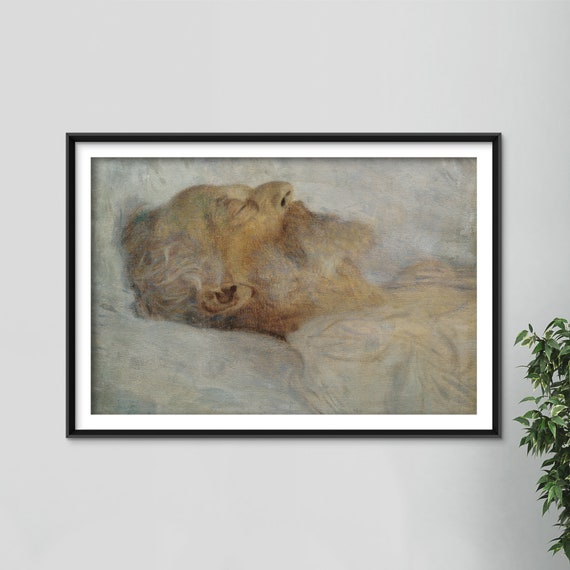This image depicts a framed painting hanging on a white wall. The painting is enclosed in a black frame with an inner white border. Adjacent to the painting, partially visible, is a fake tree with green leaves. The artwork itself portrays an elderly man lying down, possibly on his deathbed, with his head resting on a pillow. The man has white and gray hair, a whitish-gray beard, and a light brown mustache. His eyes are closed, and his facial expression appears peaceful and free of stress, suggesting he might be in his final moments. The painting is distinguished by its soft, ethereal colors and gentle brushstrokes, which lend a serene, ephemeral quality to the scene. The depiction emphasizes his advanced age, as evidenced by his large ears, curved nose, and prominent wrinkles. He appears to be wearing bedclothes or a white shirt, further enhancing the impression of him lying in bed. The overall effect is one of calmness and tranquility, capturing the quiet dignity of an elderly man in repose.